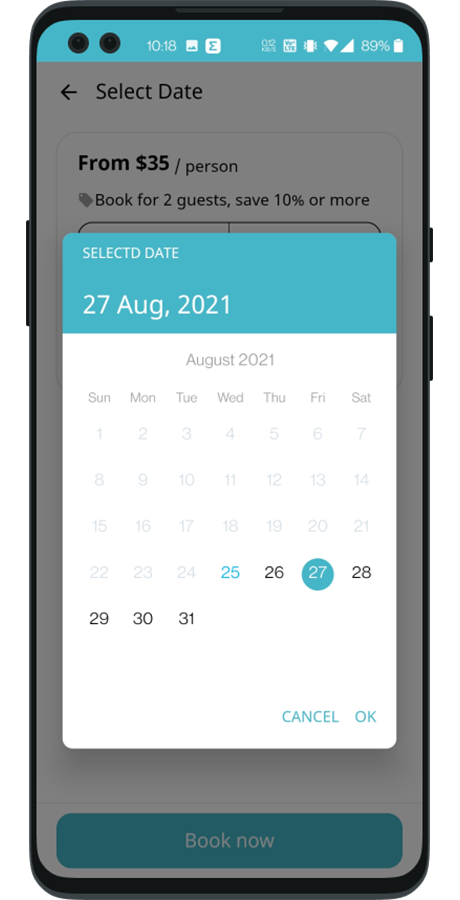The image depicts a cell phone with black borders. On the left side of the phone, a large button is visible, likely for volume control. On the right side, there are two smaller buttons; the top one is smaller than the bottom one. 

At the top of the screen's display, two black circles are situated in the middle. Adjacent to these circles is the time display reading 10:18. There are various icons including a picture icon, another unidentified icon, a toggle icon, a WiFi signal icon, and a cellular signal icon. The battery icon shows a charge of 89%.

Beneath the icons, the screen displays "Select Date" followed by a left-pointing arrow. Below this text, there's a promotional message: "From $35 a person. Book for two guests. Save 10% or more", accompanied by a coupon icon.

Part of the screen shows an overlay for selecting dates in August, but there is a typographical error where "SELECT DATE" is spelled as "SELECTD DATE". The specific date highlighted is "27 August 2021". This is further emphasized with a white background section that reads "August 2021" with "Friday the 27th" highlighted in blue. At the bottom of this section, there are two buttons labeled "Cancel" and "OK".